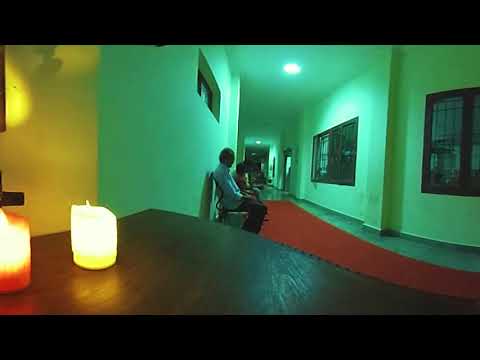The photograph depicts a long, dimly lit hallway painted in a bright green color, which is given a greenish hue by the lighting. The floor is adorned with a long, dark red rectangular rug that runs down the middle. To the right, the hallway features two large windows and an open doorway, with a smaller window visible in the distance. On the left side of the hallway, a row of people sits in chairs against the wall, beneath a small, barred window.

In the foreground, occupying the left third of the image, there is a wooden table. On top of the table, two lit candles—a yellow one and an orange one—are positioned, casting a warm, white light with hints of red and yellow, which illuminates the scene. The overall setting appears to be a communal space, with the hallway extending into the background, showing additional ceiling lights that are dimmer and ineffective in brightening the room.